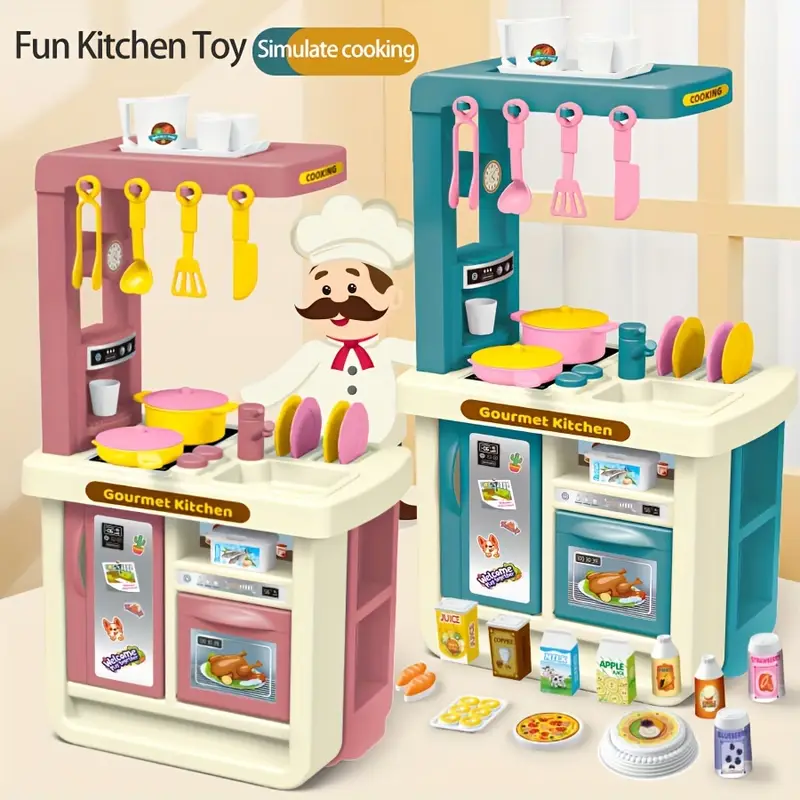This image features a detailed and colorful depiction of a children's kitchen toy set. In the top left corner, the text "fun kitchen toy" is prominently displayed, followed by "simulate cooking" within a rounded rectangle that transitions from a greenish-blue background to an orange one. The scene showcases two toy kitchen stations, each designed with inverse colors: the left one is pink with a white countertop, accented by yellow pots, utensils, and dual-colored plates, while the right one is bluish-green with a white countertop, featuring similar accents in complementary colors. Both kitchen sets are labeled "Gourmet Kitchen" on the front. A little chef figure, seemingly male, stands between the two stations. The toy kitchens are equipped with sinks, burners, refrigerators, ovens, and coffee makers, complete with playful illustrations of food items. The floor in front of the bluish-green station is scattered with various toy food boxes, adding to the vibrant and engaging setup.